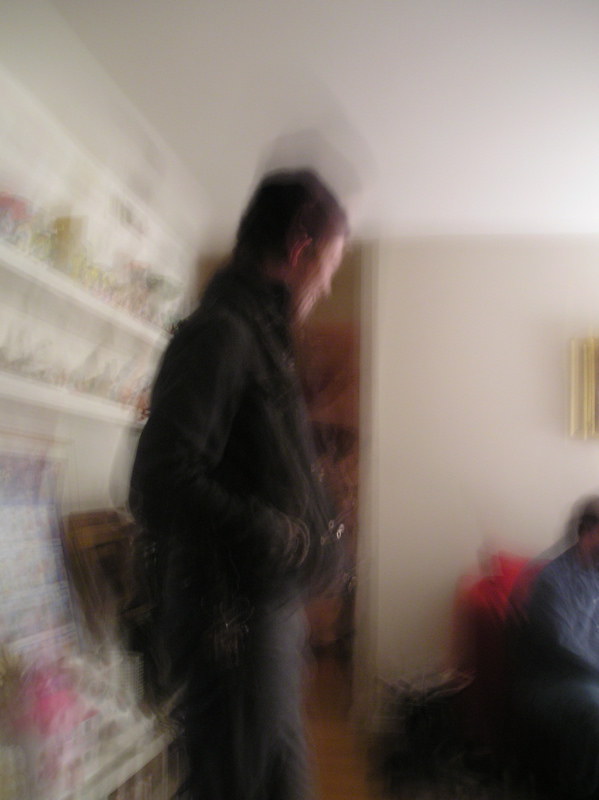In the image, an out-of-focus scene depicts a man standing in a living room. The man, wearing gray pants and a brown jacket, appears to have keys in his pocket. He has short brown hair. Another person is seated on a couch in the bottom right corner of the scene, seemingly observing the activity on the couch. The background features a white wall, and to the left, another wall showcases a couple of mantles adorned with indistinct items. A bin, possibly containing pictures, is also visible to the left. Beyond the focal point, there is an opening leading to another room.